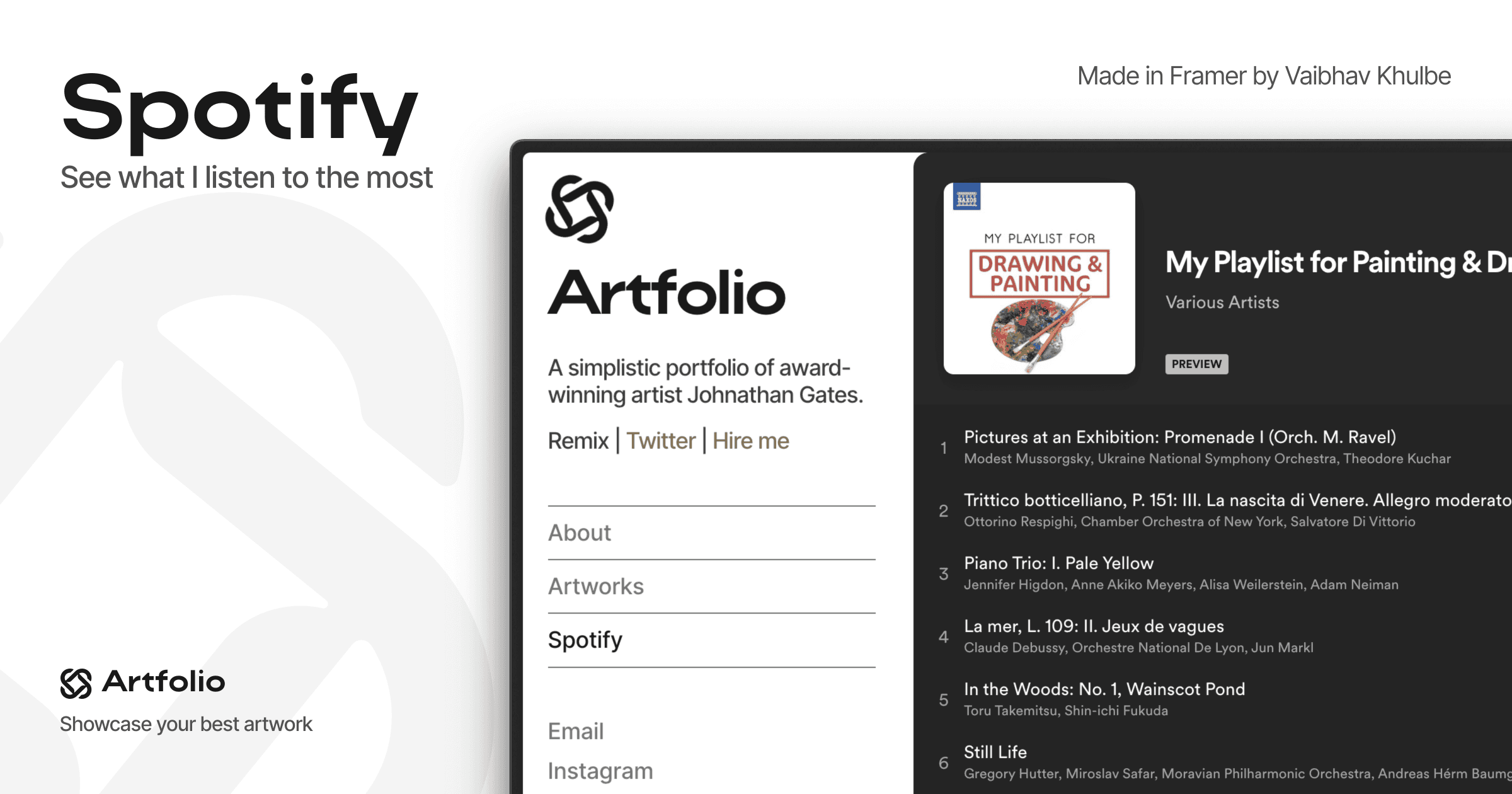The image depicts a web page featuring a blend of content from Spotify and Artfolio. In the upper left-hand corner, the Spotify logo is prominently displayed in black text. Beneath the logo, in smaller font, the text reads, "See what I listen to the most."

In the upper right-hand corner, there is dark gray text that states, "Made in Famer by Viabhav Khulbe." This suggests some affiliation or recognition within the platform.

Moving to the bottom left-hand corner, there is the Artfolio logo accompanied by the company's tagline, "Showcase your best work." This portion signifies that the main focus of the page is related to Artfolio.

Central to the page, "Artfolio" is written in bold black text, followed by the description, "A simplistic portfolio of award-winning artist Jonathan Gates." Underneath this description, there are clickable options for "Remix," "Twitter," and "Hire Me," arranged horizontally.

Vertically aligned beneath these options, there are links labeled: "About," "Artworks," "Spotify," "Email," and "Instagram." These links provide navigation through different sections of Jonathan Gates' portfolio.

On the right side of the page, with a black background, there's information about a specific Spotify playlist: "My playlist for drawing and painting" – highlighting the artist's curated music collection for creative activities. This indicates that the page showcases Jonathan Gates' portfolio alongside his personal Spotify playlist, integrating his musical tastes within his professional showcase.